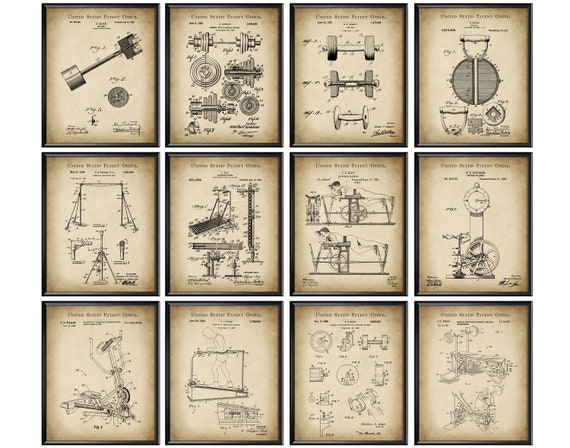This image showcases 12 intricate, antique-style diagrams of automotive components, likely designed for patent filings. Arranged in a grid with four diagrams per row, each one is framed with a dark brown border, and the overall paper has a sepia-tone that darkens at the edges, suggesting age. The top row features four diagrams: the first on the left appears to be an automobile piston with a metal object and a handle; next to it are sketches of circular metal objects and brakes. Continuing right, the third diagram shows three metal objects with handles, likely related to the back axle system with wheels flanking each side. In the middle row, diagrams detail other significant automotive parts, including an A-frame structure, piece by piece. Among these, one depicts a person partially reclining on a table, likely illustrating the assembly process or part usage. All texts in the diagrams are too diminutive to read, contributing to the vintage aesthetic and lending an air of technical craftsmanship.